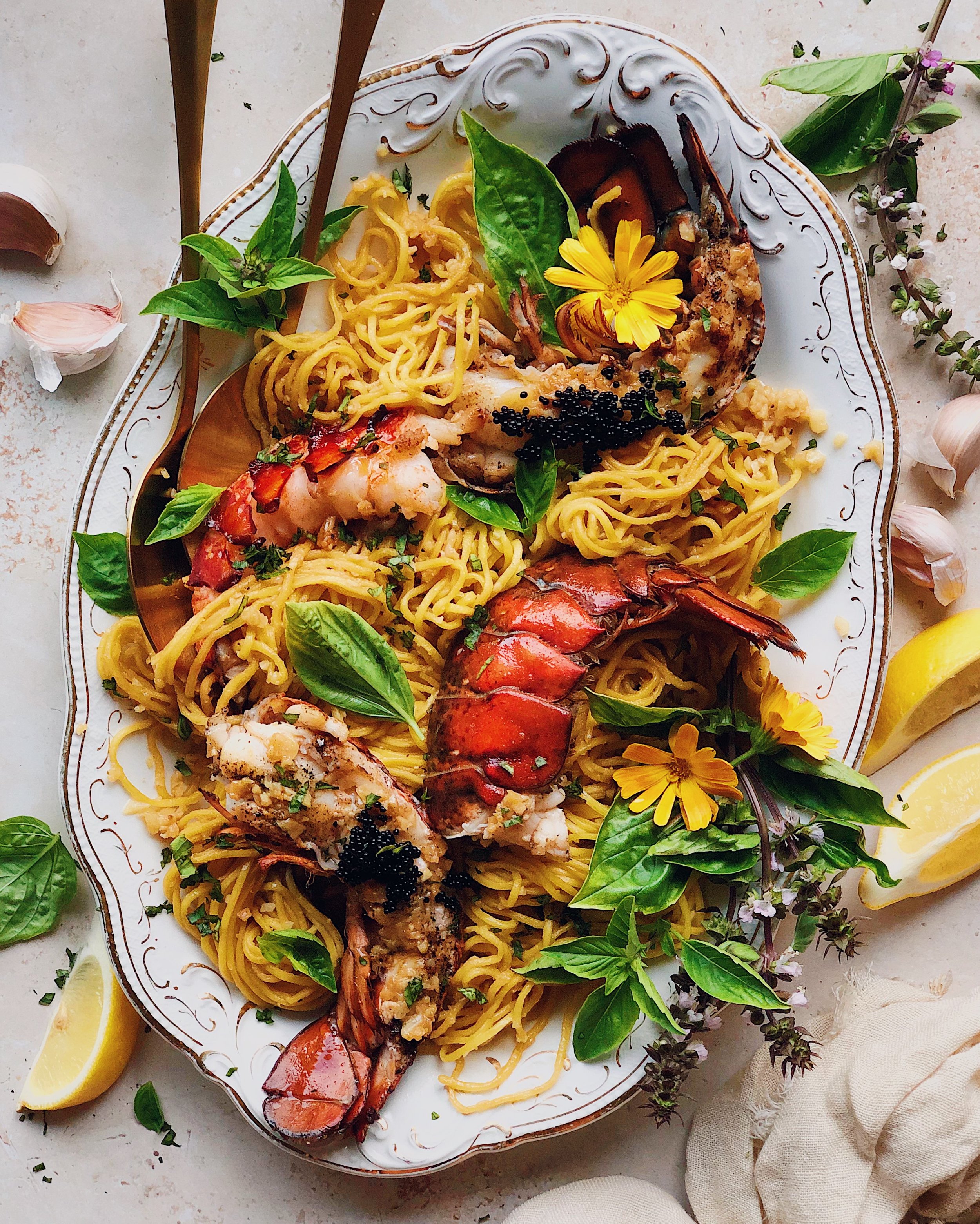In this indoor image, set against a grayish-white background, a long, oblong serving dish with ornate gold decorations and a gold rim takes center stage. The dish is filled with a sumptuous pasta and seafood combination. Nestled within a generous serving of yellow-hued noodles are well-cooked lobster tails, still in their shells, and sprinklings of caviar. The meal features garnishes of fresh basil leaves, lemon wedges, and sprigs of parsley, along with a couple of buds of delicate yellow flowers for decoration. Scattered around the white linen-covered table are various elements including tiny flower branches, unpeeled garlic cloves, additional lemon slices, and a cloth. Two elegant gold spoons are ready to serve this enticing dish, making it a feast for both the eyes and the palate.